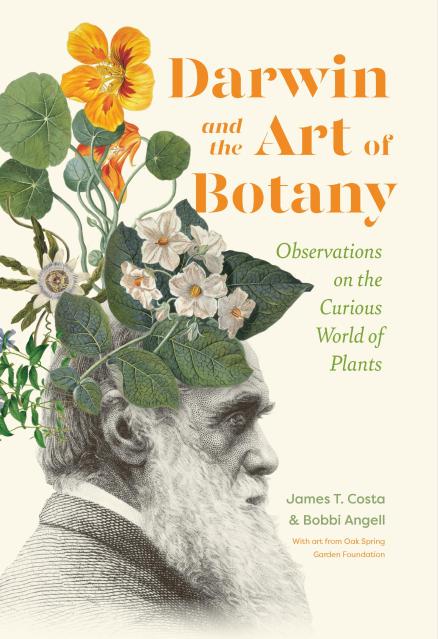The book cover features an off-white beige background with the title "Darwin and the Art of Botany" prominently written in large, orange, right-aligned font at the top right corner. Just below, in smaller green text, is the subtitle "Observations on the Curious World of Plants." The authors' names, James T. Costa and Bobby Angel, are displayed in small green text at the bottom, followed by a note in tiny orange text that mentions "With Art from Oak Spring Garden Foundation."

On the left side of the cover, a detailed black and white sketch, or photorealistic drawing, portrays an elderly Charles Darwin with a long white beard and gray hair. He is depicted wearing a suit jacket made of stiff formal material over a white undershirt. On Darwin's head, there are colorful illustrations of various flowers and leaves. The top set of leaves are rounded, while the ones below are football-shaped. The flowers include both white and orange blossoms, adding vibrant contrast to the monochrome sketch beneath them.